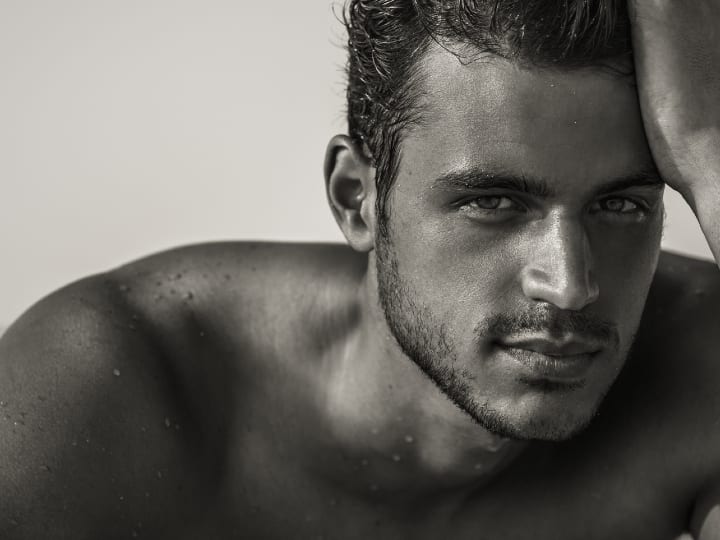This black and white close-up photograph captures a shirtless male model against a light gray background. The model, positioned with his shoulders visible in the bottom half of the frame and his head slightly to the right, exudes a chiseled and intense look. His short, wavy dark hair complements his relatively light skin and prominent dark eyebrows. He gazes directly at the camera with light-colored irises, adding to the intense vibe of the portrait.

The model's facial hair includes a faint mustache and a stubbly beard that extends into a chin strap. His left hand is held up against his forehead, with his palm visible, emerging from the top right off-frame. Small beads of liquid are noticeable on his muscular shoulders, neck, and face, suggesting he might have just come out of water, adding a sense of refreshment to the composition. The very bottom of the frame is slightly blurred, focusing attention on his upper body and facial features. Despite the black and white format, the image hints at his naturally tan complexion. His lips are pressed together in a slight smile, though no teeth are shown, further enhancing the intense and sophisticated aura typical of a high-fashion or cologne advertisement.